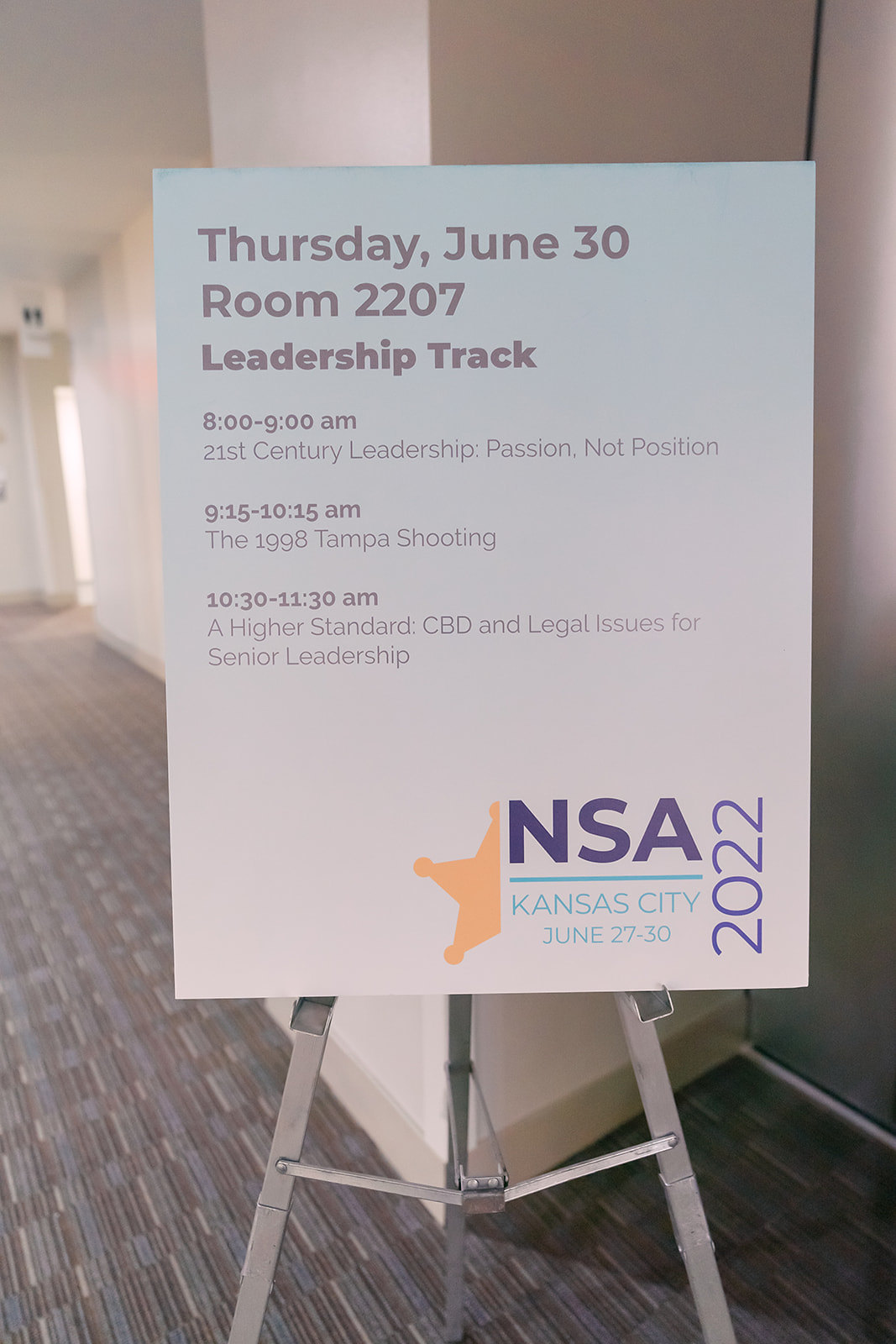The image depicts a silver easel stationed in a long, relatively empty hallway with off-white walls and carpet laid out in a gray and blue pattern resembling bricks, angled off at approximately a 10:30 direction. The prominent feature on the easel is a large, white poster providing details about a conference event. The heading at the top of the poster reads "Thursday, June 30th, Room 2207," followed by "Leadership Track" in dark lettering. Detailed schedule entries are listed below: "8 to 9 a.m. – 21st Century Leadership: Passion, Not Position," "9.15 to 10.15 a.m. – The 1998 Tampa Shooting," and "10.30 to 11.30 a.m. – A Higher Standard: CBD and Legal Issues for Senior Leadership." In the lower right corner of the poster, there is a logo featuring a half-star emblem and the text "NSA 2022" in purple, "Kansas City" in blue, and the dates "June 27th to 30th" all in light blue, indicating the event's host and location.